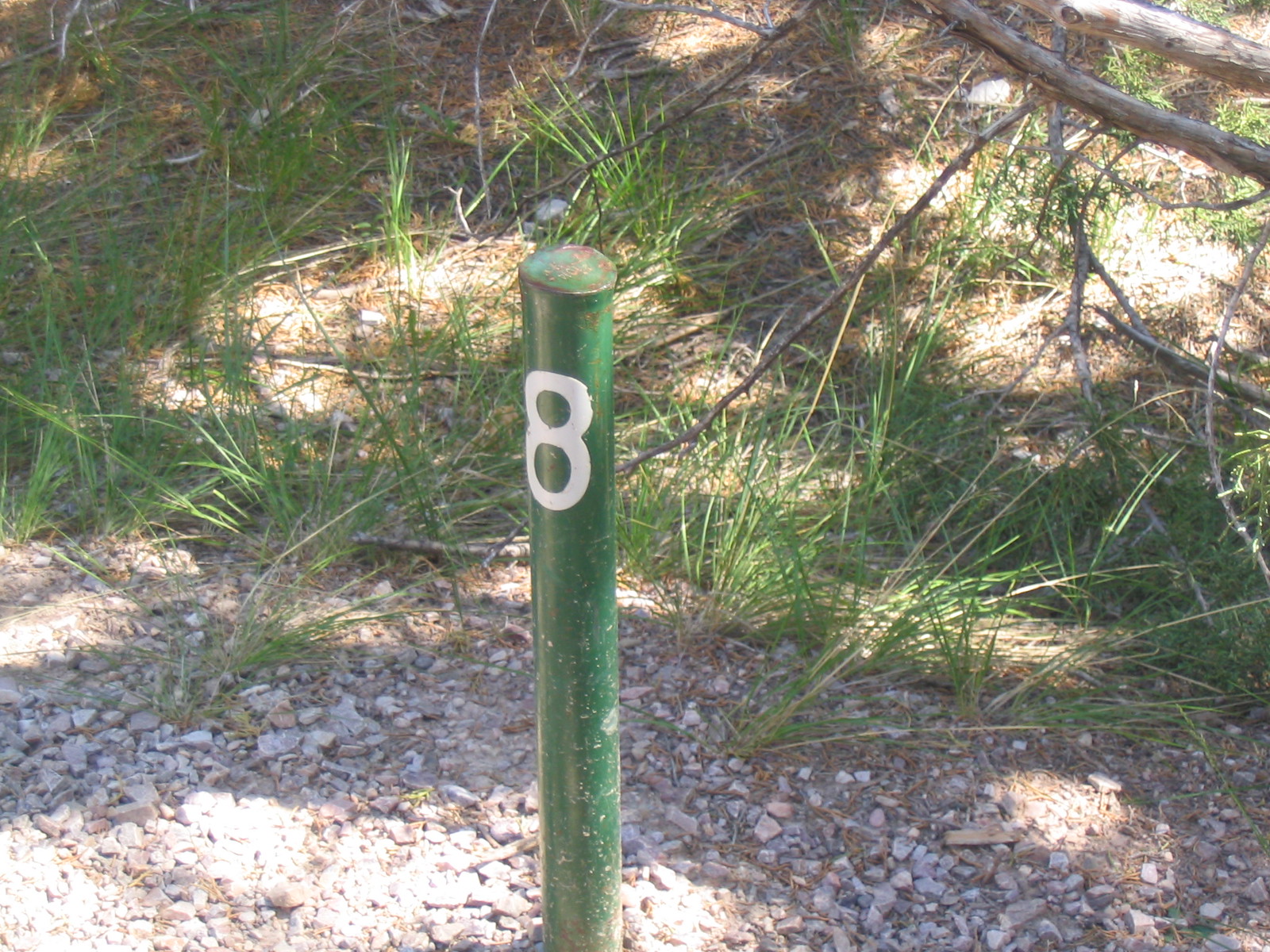This outdoor photograph features a central cylindrical green-painted metal pole exhibiting signs of rust, especially near the top. The pole, which stands prominently from the bottom center to just above mid-frame, has the large number 8 painted vertically in white near its upper section. Surrounding the pole, the ground is a mix of stony terrain and patches of weeds, grass, and scattered pebbles. The top right corner of the image is marked by two light and dark brown branches, likely from a dead tree, with a few green pine needles protruding from slender stems. Additionally, the background hints at a slight elevation in the terrain, with occasional long plants dotting the otherwise rocky and dirt-laden ground.